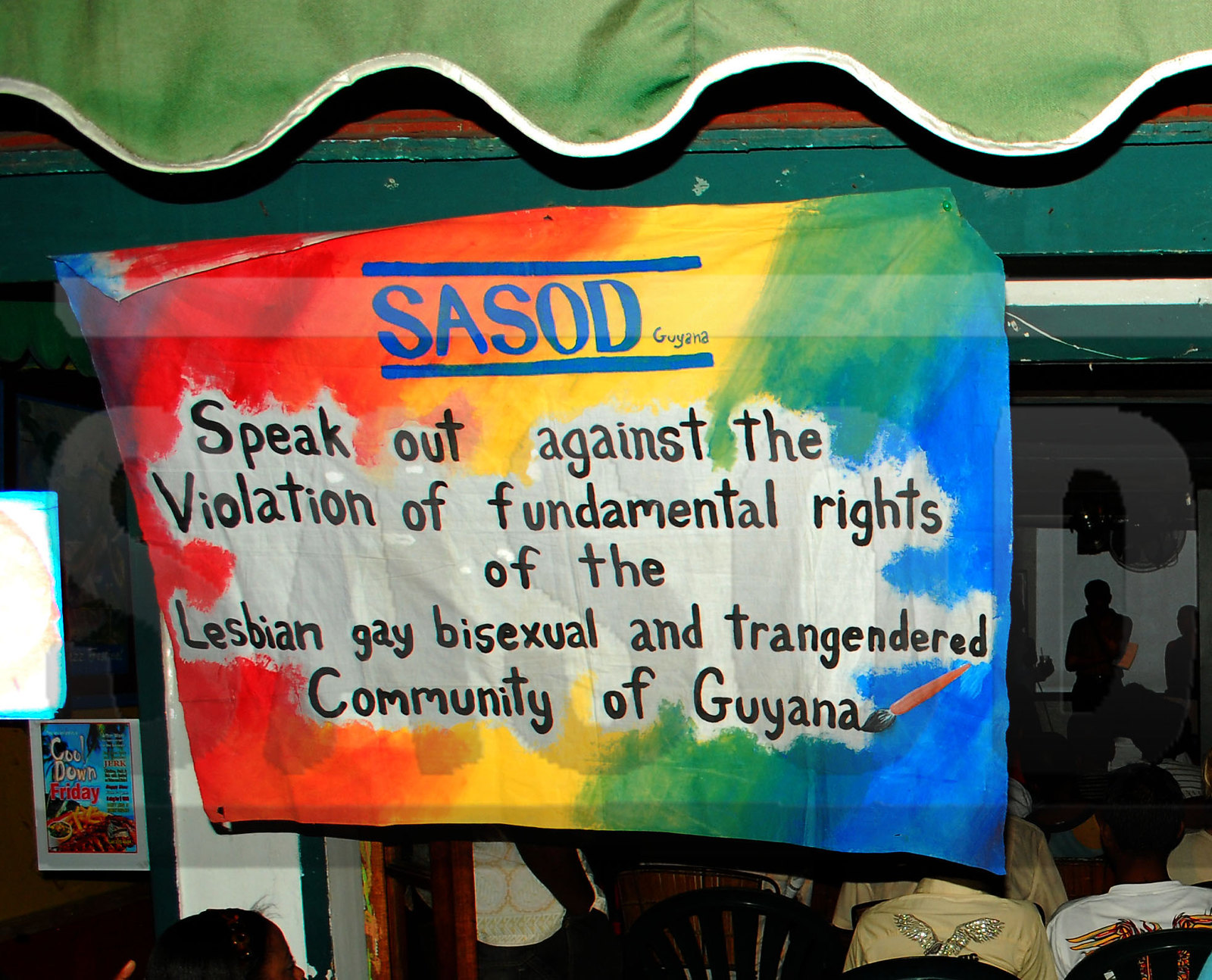The image features a vibrant outdoor scene focused on a brightly colored rainbow banner hanging prominently in the center. The banner, rectangular and brightly splattered with red, green, yellow, blue, and other rainbow colors, boldly declares in black ink: “SASOD Guyana - Speak Out Against the Violation of Fundamental Rights of the Lesbian, Gay, Bisexual, and Transgendered Community of Guyana.” The banner is affixed to a wooden shelf, just beneath a green cloth with a white hem, crafty cut in a wave shape. The setting appears to be outside of a restaurant or community gathering area, with the lively scene augmented by a crowd visible to the right, seated in chairs and watching an unseen speaker. To the left, a smaller sign reads "Cool Down Friday," adding context to the event. The overall mood is one of activism, solidarity, and support for LGBT+ rights, highlighted by the myriad colors symbolizing inclusivity and pride.